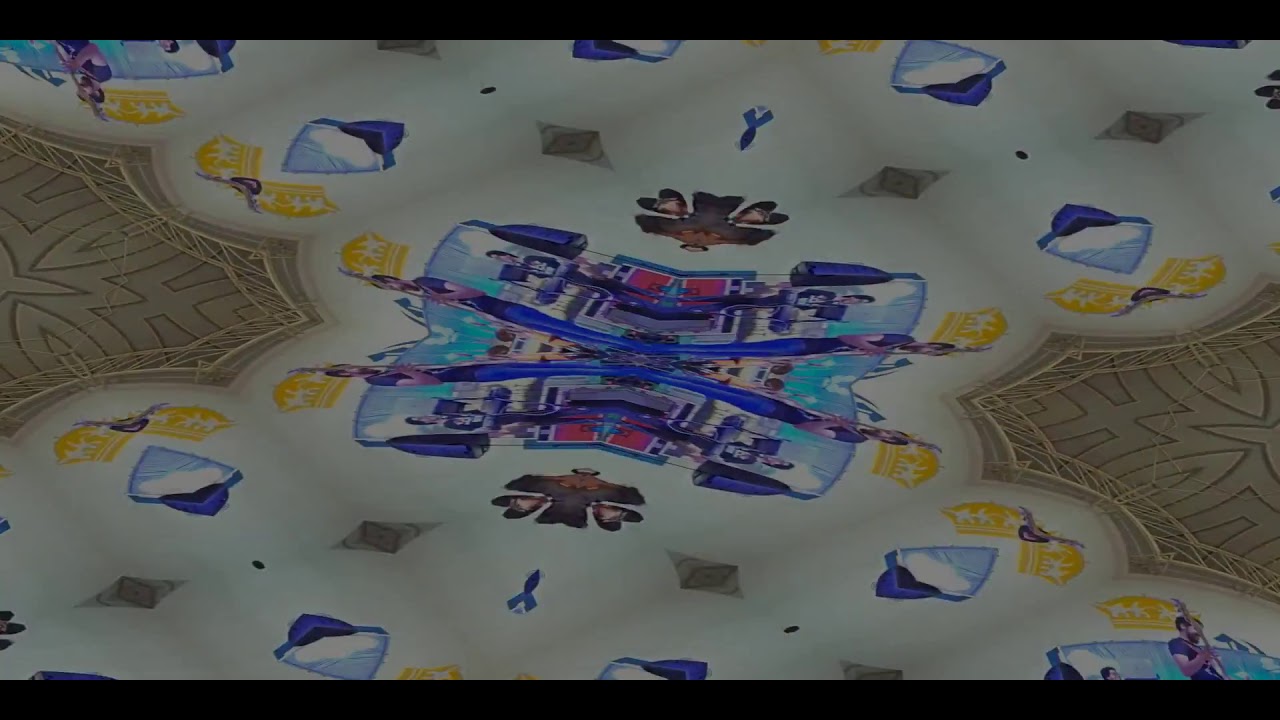This intricate image appears to be the result of a kaleidoscopic or mirrored effect, creating a mesmerizing design that radiates from the center. Central to the composition is a distorted, repeated image of a man wearing blue pants and a dark blue shirt, holding a guitar. The man's likeness is reflected multiple times across the image, appearing in repeating quadrants with two on either side and additional reflections at the top left and bottom right corners.

The background is richly detailed with several recurring elements, including a schematic network in blue and red shades, parallel lines, and an array of geometric and organic shapes. Noteworthy features include a blue-shaped bulb, a guitar pick-like object with a purple, blue, and white melange, some of which contain small heart shapes. An ethereal, gray moth with heart-shaped wings is distinguished in a plus structure. Dark gray rectangles and yellow-starred patterns add further complexity, while subtle brown patterns flank the sides, completing the elaborate and visually compelling scene.